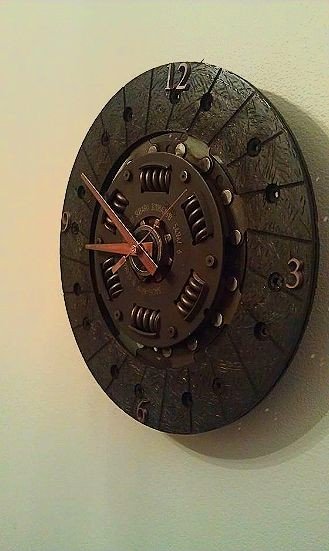This is a detailed color photograph of a distinctive, dark brown, custom-built wall clock that exudes a steampunk aesthetic. The clock is hanging on a cream-colored wall, casting a shadow to the right. The analog clock prominently features the numbers 12, 3, 6, and 9 rendered in a lighter, copper-toned metal, while the remaining numbers are absent. The clock's round frame appears to be constructed from a metallic material with intricate detailing, including six visible springs set into a secondary circle around the center. The most central point of the clock displays a metal gear, contributing to its mechanical appearance. The clock's hands are a worn red color, with the short hand just below the 9 and the long hand above the 9. Additional decorative elements and screws adorn the clock, enhancing its vintage, mechanical look. The combination of the cream wall and the clock's dark tones make it a striking focal point in the photograph.